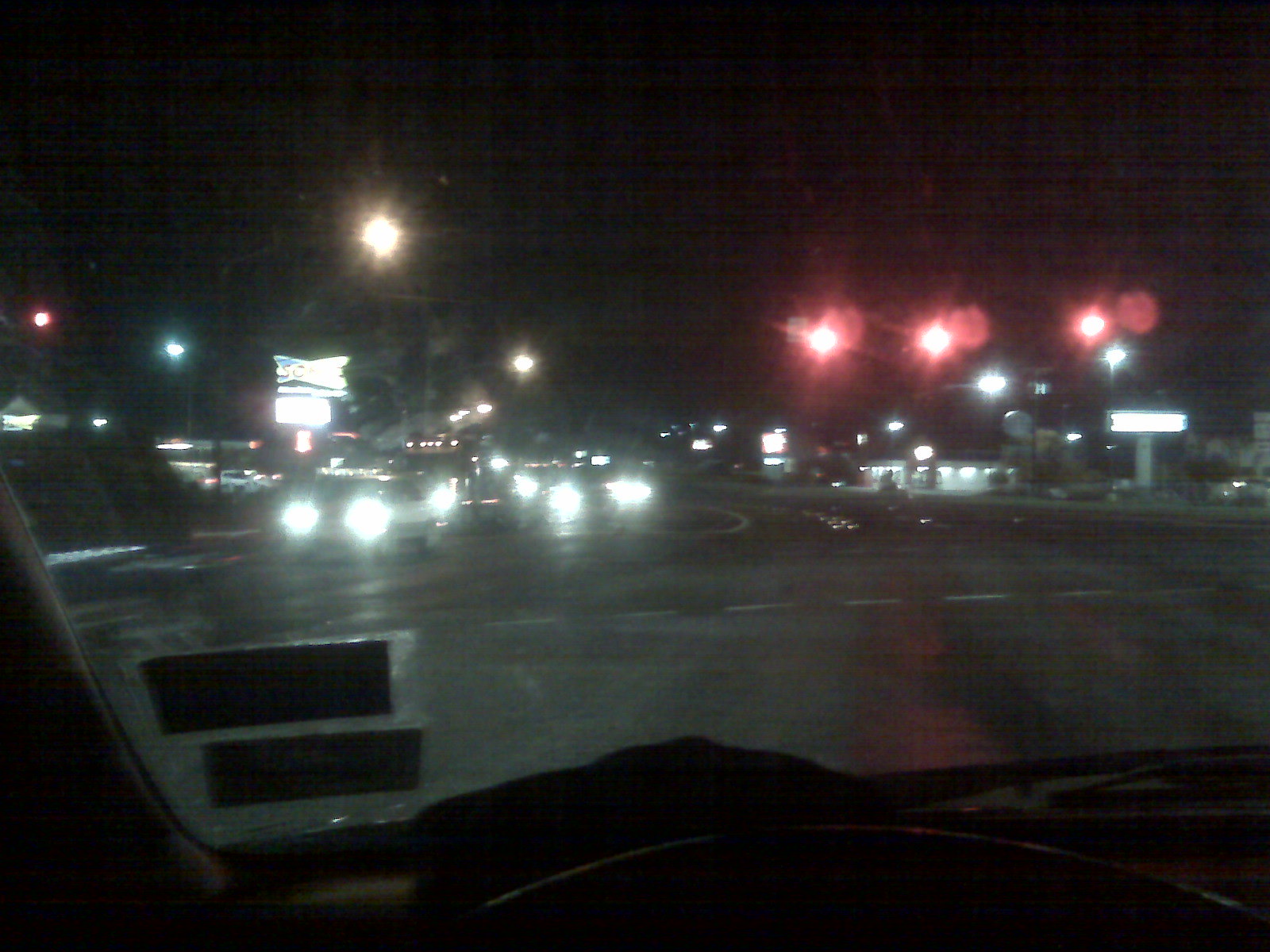The photograph captures a nighttime street view from inside a vehicle. The car's interior is subtly visible at the bottom of the image, with a dark, shadowy area indicating the dashboard and two rectangular stickers faintly outlined at the bottom left corner of the windshield. Through the windshield, the road stretches ahead, illuminated by streetlights. Suspended from a pole above the road, a traffic light displays three glowing red signals. In the distance, beyond the traffic light, a store front radiates light, creating a warm contrast against the dark night. On the left-hand side of the road, multiple cars are driving towards the viewer, their headlights piercing through the darkness. Further in the background to the left, a brightly lit establishment, possibly a Sonic restaurant, hints at activity and perhaps a place for a late-night meal. The entire scene captures the stillness and ambiance of a nighttime urban setting.